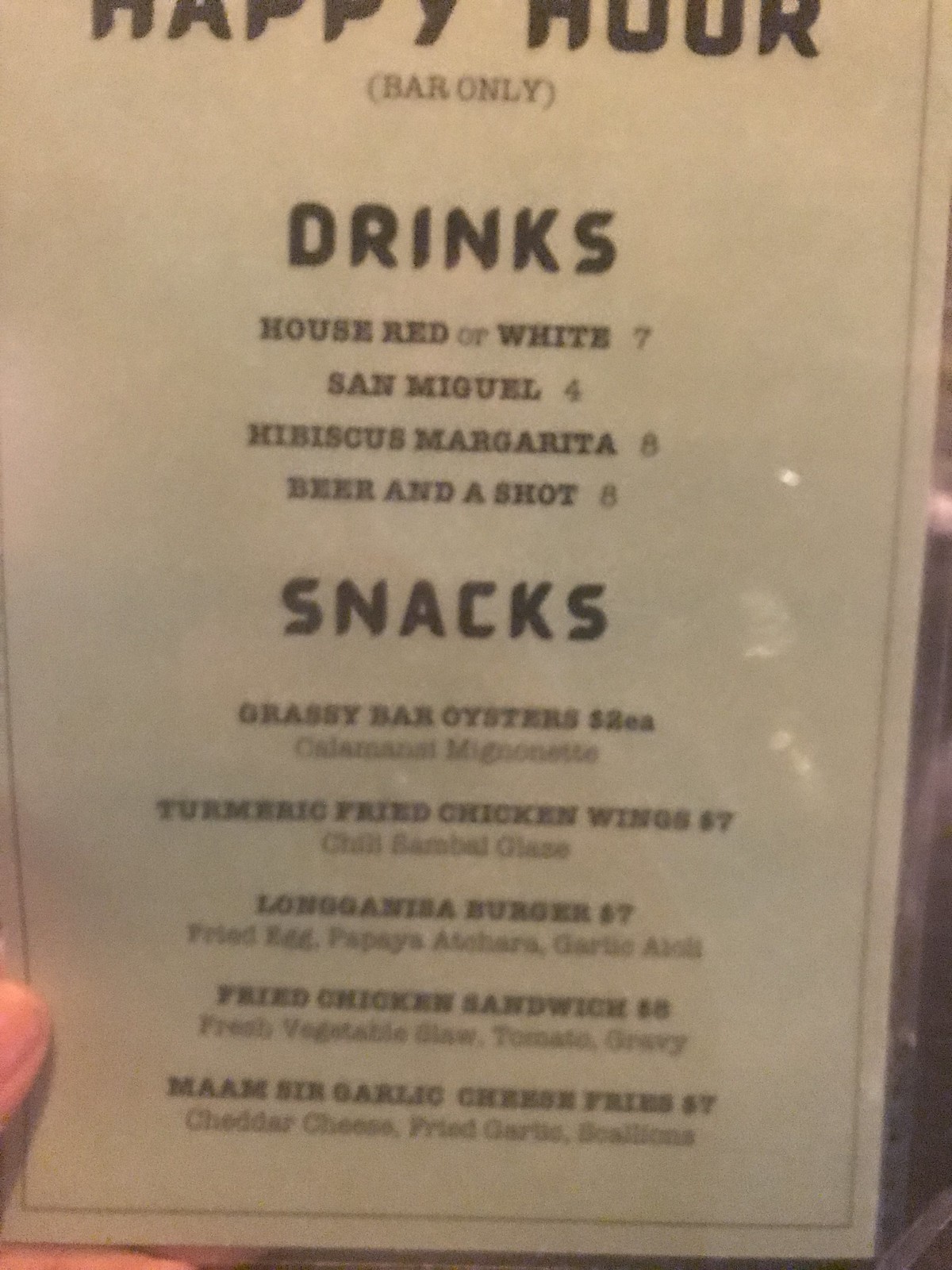This is a detailed description of a happy hour menu from a certain establishment. The top of the menu clearly states "Happy Hour" with "bar only" in brackets next to it. Below that, the section titled "Drinks" is prominently displayed in a larger font. 

The drink options listed are:
- House Red or White: $7
- San Miguel: $4
- Miss Hibiscus Margarita: $8
- Beer and a Shot: $8

Following the drinks, there's a section labeled "Snacks." The snack items are as follows:
- Grassy Bar Oysters: $2 each (noted as "EA")
- Calamansi Margarita
- Turmeric Fried Chicken Wings: $7
- Chill Season Sample Platter
- Lingui Longanisa Burger: $7
- Fried Chicken Sandwich: $8
- Manse Garlic Cheese Fries: $7

Some items may appear slightly unclear, but the provided information conveys a comprehensive list of available happy hour offerings.